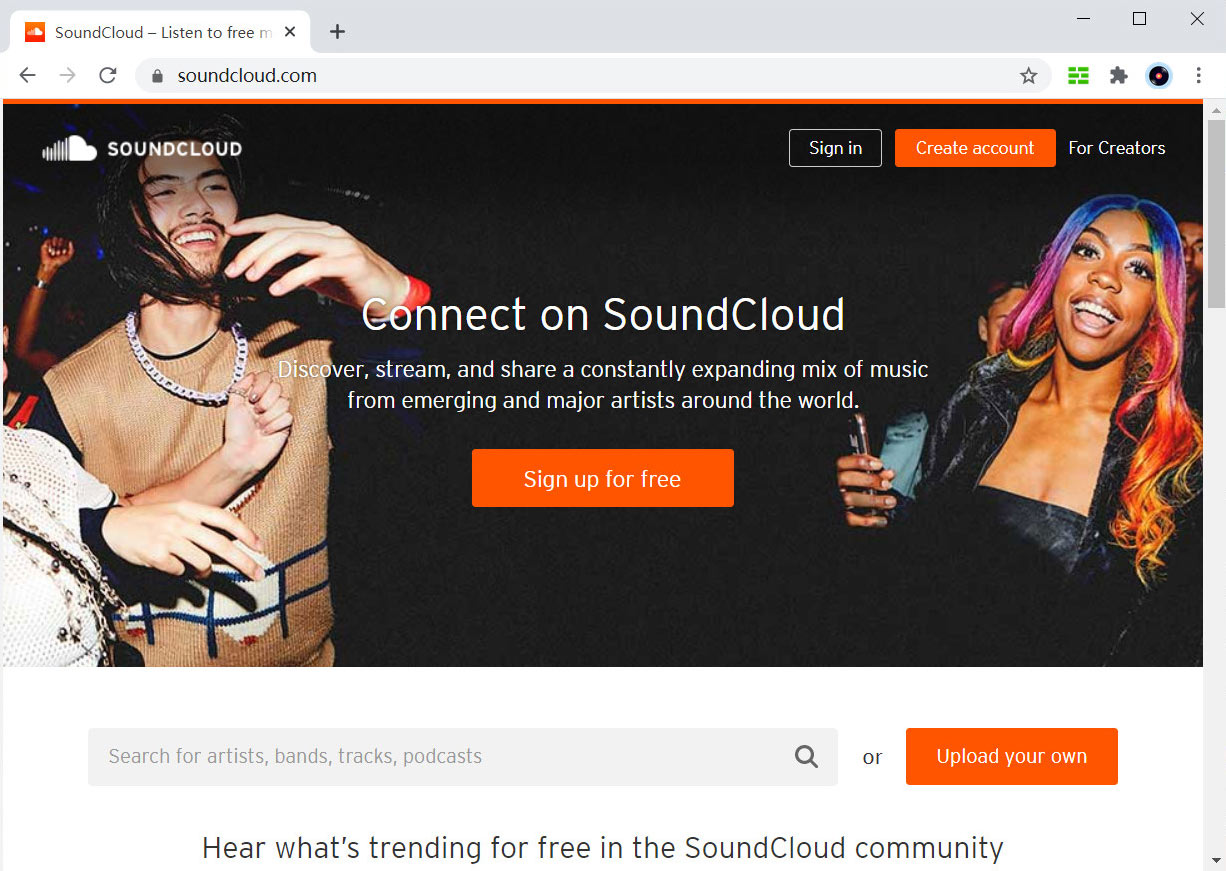This screenshot captures the interface of the SoundCloud website as displayed on either a tablet or desktop web browser. The browser tab, located in the upper left corner, reads "SoundCloud - Listen to free music," and the URL bar directly below confirms the address as SoundCloud.com.

The main body of the webpage features a black background adorned with vibrant images. To the left, a man appears to be dancing joyously, while on the right, a woman with rainbow-colored hair looks equally delighted.

In the upper left corner of the image, the SoundCloud name and logo are prominently displayed. Moving to the top right of the page, there are several interactive buttons: "Sign in," "Create account," and "For Creators."

Centrally positioned on the webpage is a bold headline that reads, "Connect on SoundCloud. Discover, stream, and share a constantly expanding mix of music from emerging and major artists around the world." Below this headline, an eye-catching orange button invites visitors to "Sign Up for Free."

Further down, a search box allows users to look for artists, bands, tracks, or podcasts. Adjacent to this search box, a prompt encourages users to "Upload Your Own" music, signifying the website's dual role as both a music discovery platform and an uploader's haven.